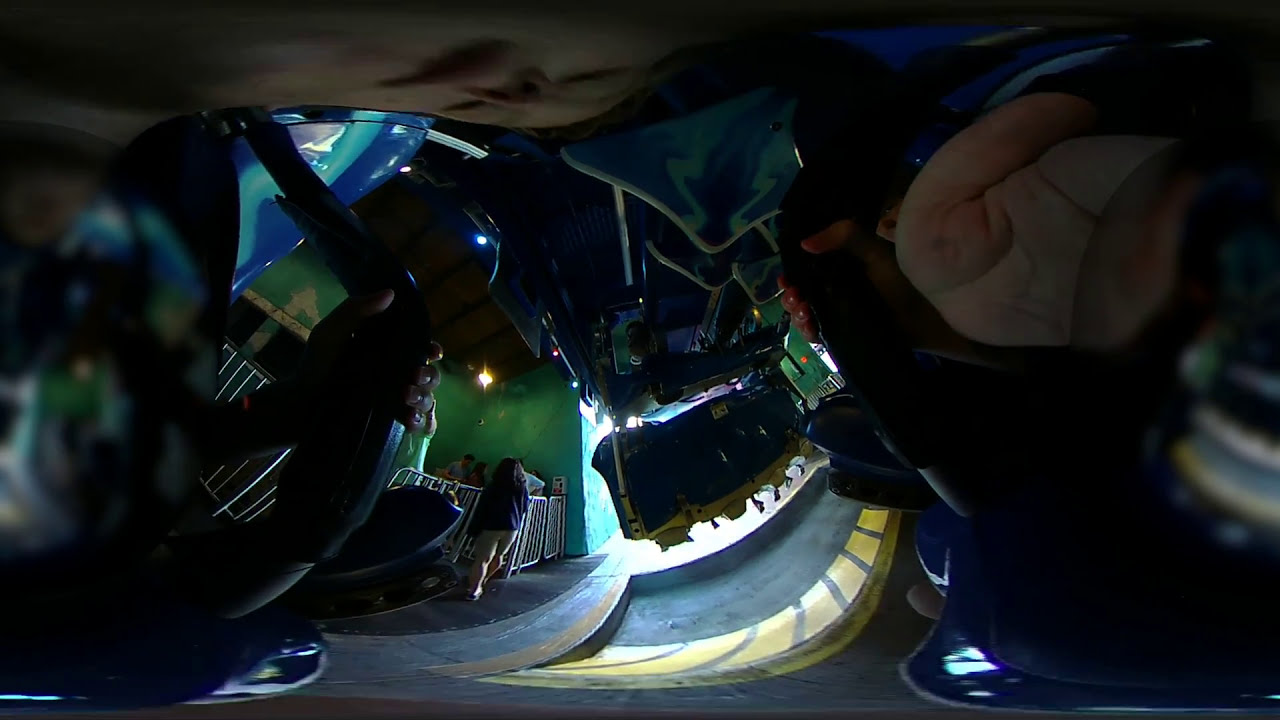This image captures the view from inside a rollercoaster carriage just before the ride begins, giving a fisheye lens effect that distorts the scene into a spiral pattern. From the vantage point, you can see the hands of riders gripping the safety bars. The rollercoaster appears to be the type where the carriage hangs, allowing feet to dangle freely. Other carriages in front of this one feature blue seats with yellow bottoms, and you can spot other riders' legs below. Directly in front, a distinct square depression in the cement floor, outlined with yellow danger markings, suggests an area for maintenance or safety mechanisms.

In the background, people stand in line, waiting for their turn. There's an attendant in the scene, facing away from the camera, near metal railings that separate the boarding area from the waiting crowd. Above, the elongated and spiraled face of the photographer appears due to the special camera effect used, adding to the surreal and dynamic feel of the image. Yellow lines on the ground may indicate paths for loaders and unloaders or guide machinery, adding to the industrial ambience reminiscent of a cargo loading area. This complex image is a blend of anticipation, industrial design, and a unique photographic twist, capturing the chaotic energy where riders prepare for the thrill of the rollercoaster.